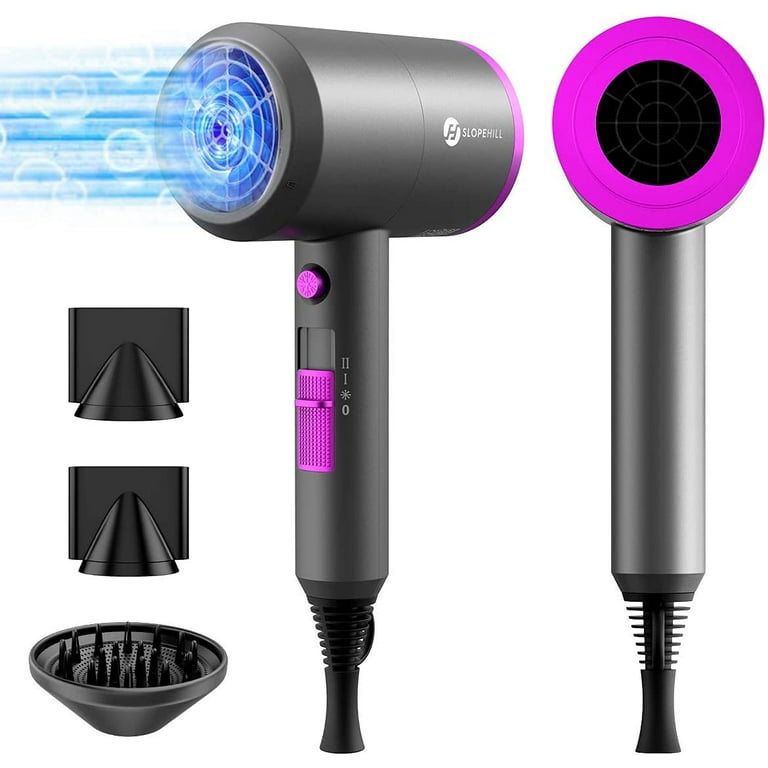This image serves as a product preview for a sophisticated blow dryer, likely intended for listing on a site like Amazon. The blow dryer is prominently featured, with two views provided for a comprehensive look.

In the foreground, the blow dryer is angled to the left, dynamically shown as active, with a digitally added wind effect illustrating its functionality. The device features a cylindrical top where the fan is housed and a perpendicular handle. A pink sliding button on the handle adjusts the settings, while a circular button with a snowflake symbol suggests a cooling option. Both the back of the blow dryer, where the fan is located, and the buttons have pink accents set against the dark gray body of the device. The brand name "Slope Hill" is displayed in white letters next to a circle icon with an "H" cut out, visible on the angled blow dryer.

To the right, a second view shows the blow dryer facing directly at the viewer, ensuring every aspect is visible. At the bottom left corner, three attachments are displayed. These include a detangling accessory with protruding bristles and two others with square bases and cone-shaped extensions, showcasing the versatility of the product.

Overall, the entire scene is set against a clean white background, emphasizing the sleek and modern design of the blow dryer.